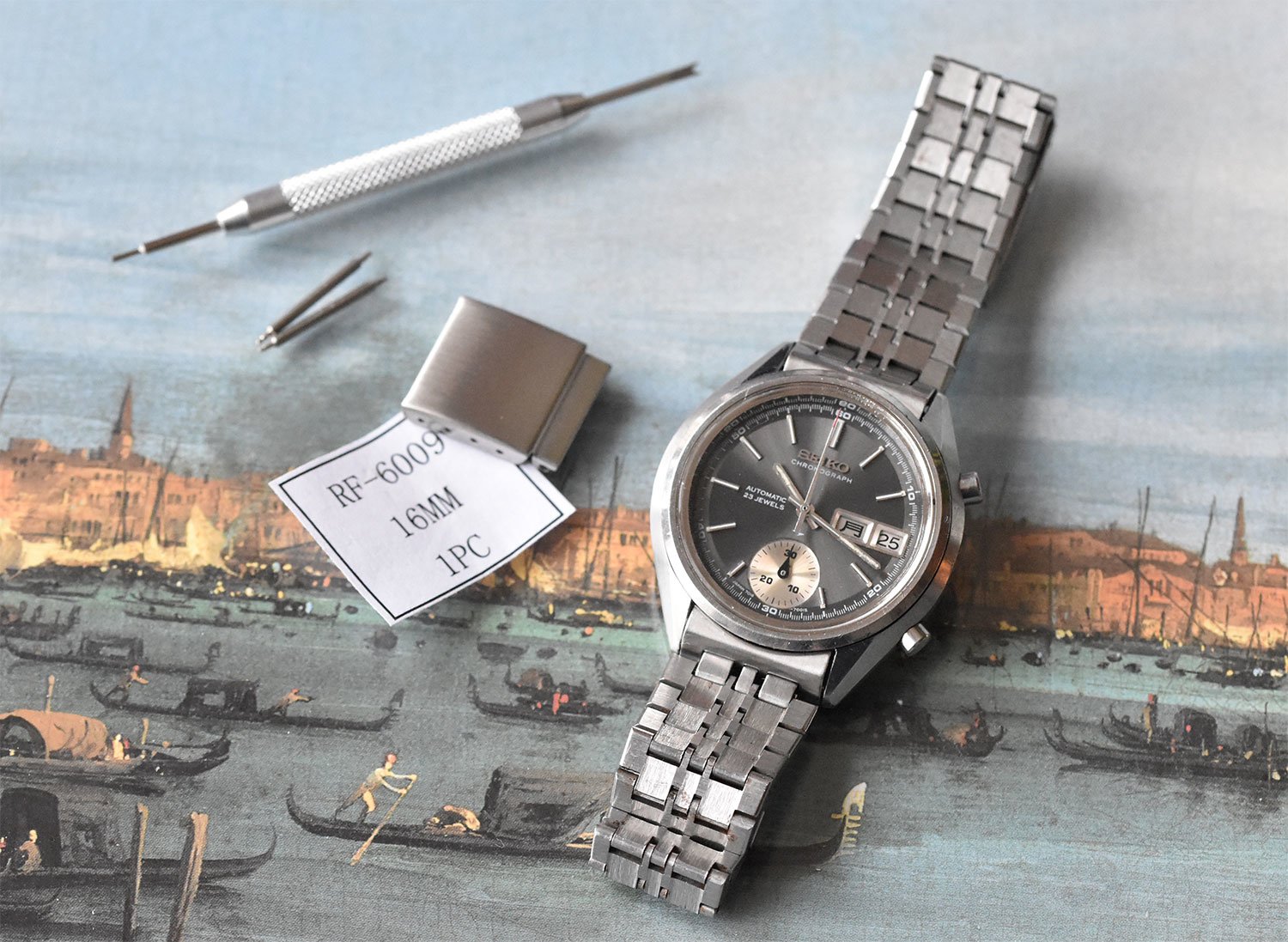The image displays a detailed close-up of a silver analogue watch with a grey strap positioned centrally towards the right. The watch sits atop an artistic painting backdrop depicting small boats with people rowing, calm waters, buildings along the shore, and a blue sky above. To the left, there are specialized watch repair tools, including a double-sided metal tool with a central grip and tweezer-like attachments. A paper tag nearby reads "RF-6009, 16mm, 1 pc." The overall scene combines the watch and its repair tools against the vividly detailed background of the painting.